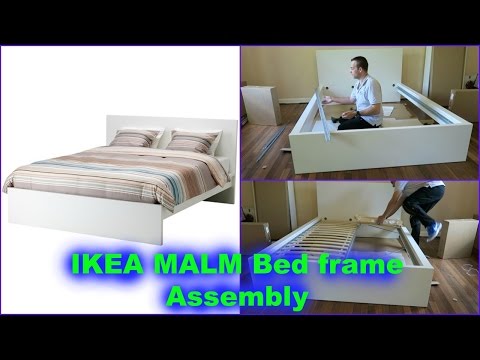The image showcases an IKEA MOM bed frame assembly in a detailed split-screen format. On the left, there are three photos displaying the fully assembled white bed frame, featuring a simple block design with a white headboard and footboard. The bed is dressed in a beige, white, and blue striped comforter, with two pillows at the end, set against a white background. On the right, two stacked images capture a man in the process of assembling the bed frame on a hardwood floor in a room with neutral cream-beige walls. In the top image, he is inside the frame, likely adjusting drawer sliders or drawer hinges while wearing jeans, a white polo shirt, and blue sneakers. In the bottom image, he is adding the supports where the mattress will rest, making significant progress in the assembly process. This detailed visual narrative appears to serve as an instructional guide or a YouTube video tutorial on assembling the IKEA MOM bed frame.